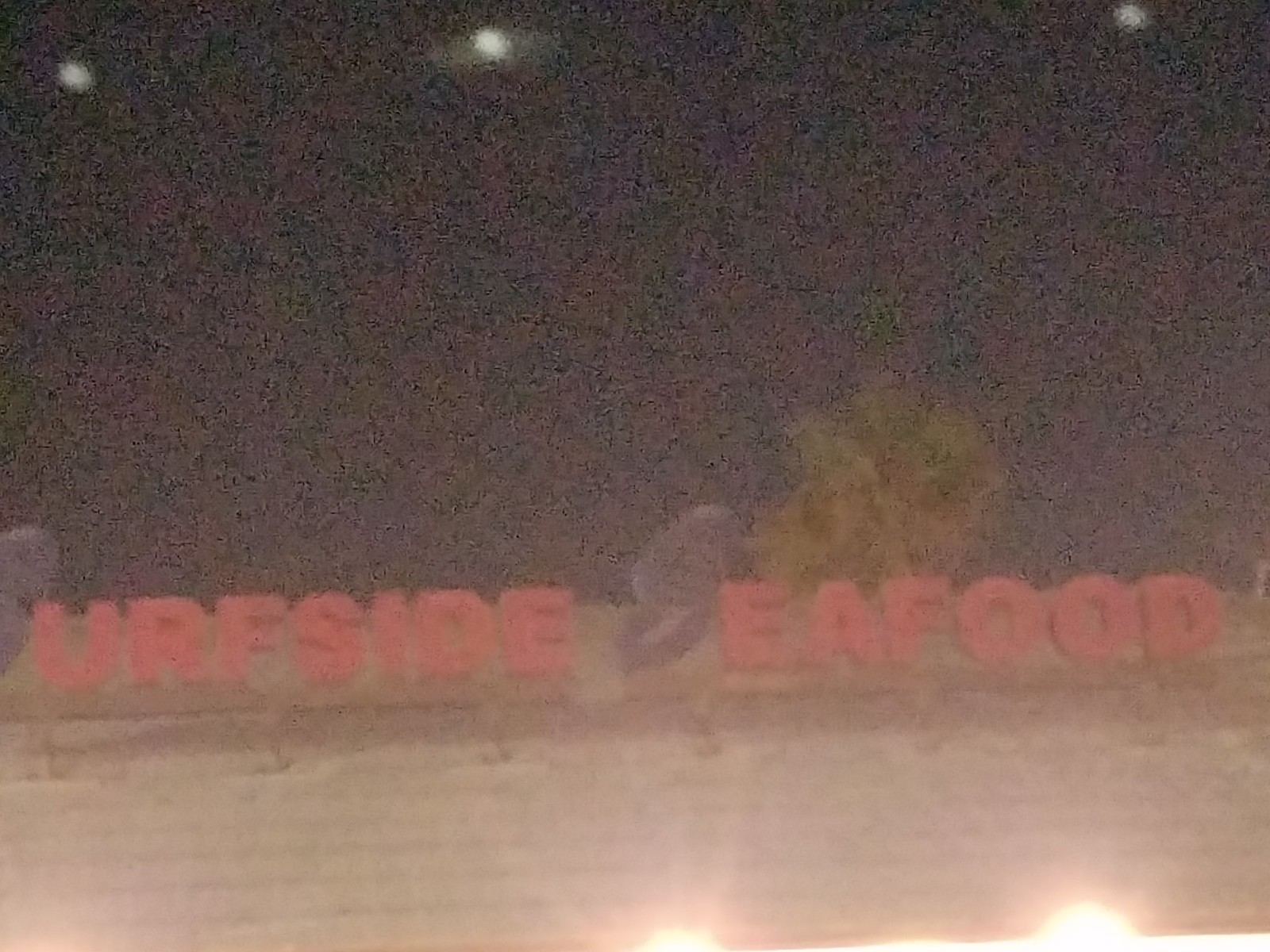A blurry nighttime photograph captures the exterior of a restaurant sign for "Surfside Seafood." The image is predominantly dark, with the top half almost entirely black, punctuated by three round white lights: one in the upper left corner, another near the middle slightly off-center to the left, and the third in the upper right corner. The illuminated restaurant sign dominates the lower portion of the image. This sign features prominently stylized gray cursive "S's" bookending uppercase red letters spelling out "URFSIDE EAFOOD." The sign is affixed to a tan brick building, with visible brackets supporting it. Above the word "Seafood," the top of a green tree is faintly visible, while the lower right-hand side of the image shows additional round lights.